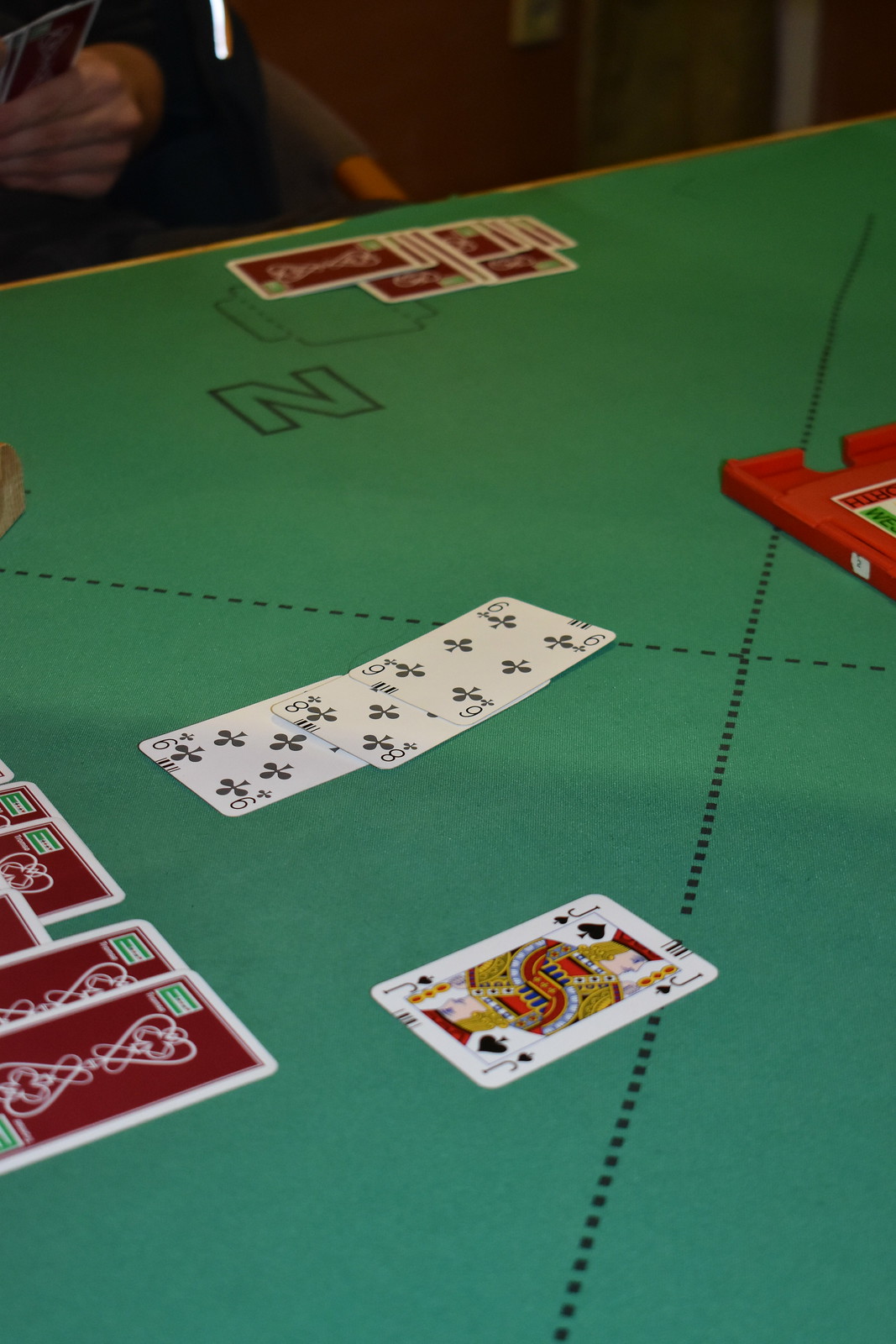This photograph, taken in portrait orientation, showcases a green gaming table, typically used for playing cards, in an indoor setting with low lighting. The table's surface dominates the image, featuring a dotted black line pattern on the right side and running horizontally across the table. Toward the back, the letter "N" is prominently displayed in block lettering on the table. Behind the table edge, the background is quite dark, suggesting a dimly lit environment. A figure or possibly a chair is faintly visible, hinting at a potential player's presence.

Positioned at the back of the table is a hand of cards, all face down, presumably ten in total. In the center of the image, three face-up cards are partially overlapped: the six of clubs, the eight of clubs, and the nine of clubs. Closer to the foreground, the jack of spades is positioned face-up at the center bottom.

To the bottom left of the image, several more playing cards are seen face down. These cards have burgundy backs with a white pattern and a small green rectangle in the top left corner. A red tray, possibly used for holding cards, peeks into the image from the right side, just above the center. The detailed arrangement of elements suggests a paused or anticipating moment in a card game.